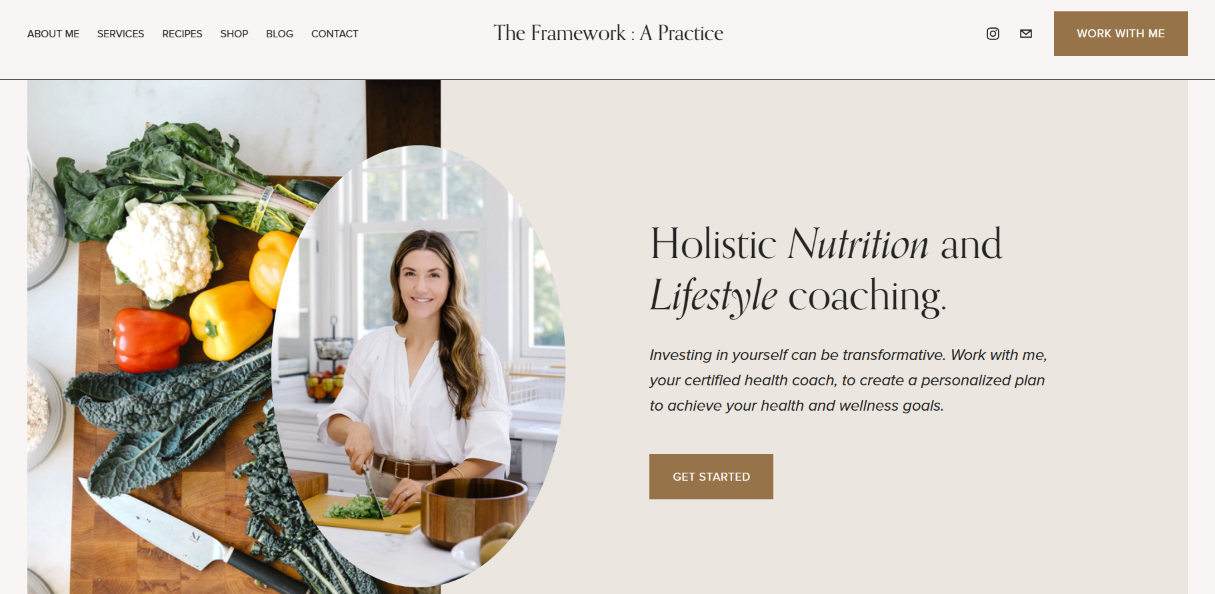This image showcases a visually appealing website with an organized layout. At the top left, a navigation menu includes links to "About Me," "Services," "Recipes," "Shop," "Blog," and "Contacts." Centered at the top, the section "The Framework, The Practice" is prominently displayed. In the top right corner, a "Work With Me" link is positioned alongside an Instagram share button and a mail icon, situated to the left of the "Work With Me" link.

The focal point of the website features a picture of a smiling lady in a kitchen setting, actively chopping vegetables with a knife. She wears a brown belt around her waist, complementing the overall aesthetic. The background of the website is a warm, light brown hue, creating a cohesive, inviting atmosphere.

To the right of the image, an engaging caption reads: "Holistic Nutrition and Lifestyle Coaching. Investing in yourself can be transformative. Work with me, your certified health coach, to create a personalized plan to achieve your health and wellness goals. Get started." This call-to-action encourages viewers to take the first step towards improving their health and wellness by collaborating with a certified health coach.